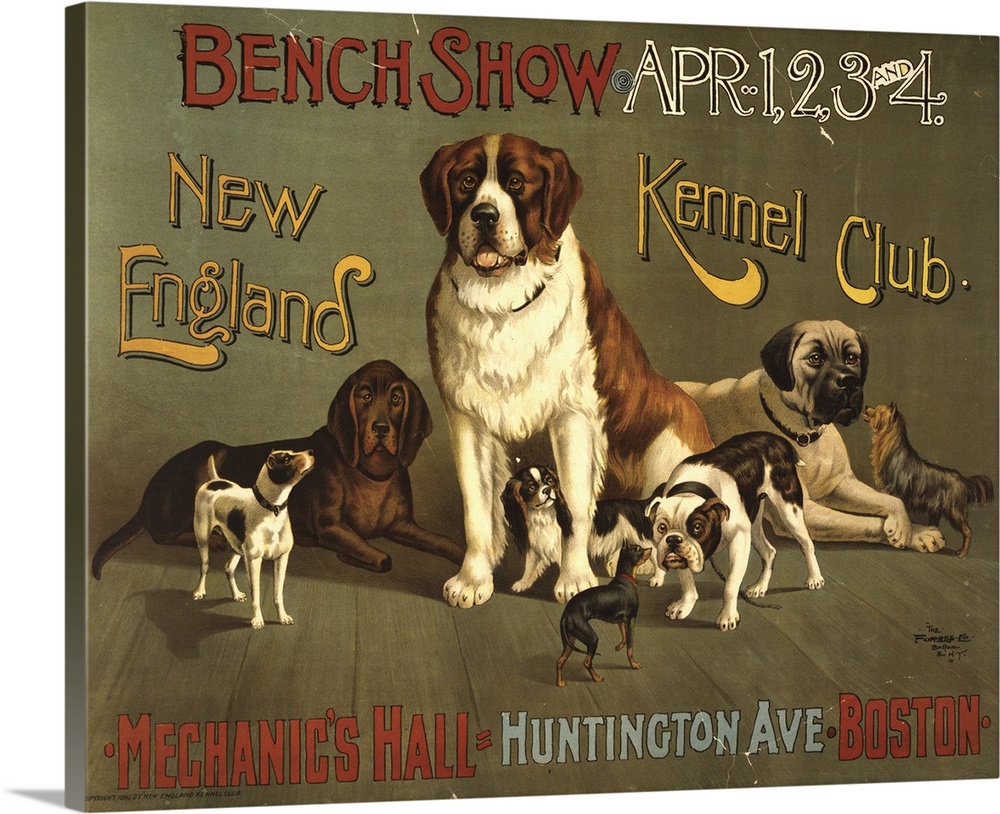This is a detailed, hand-drawn poster advertising the "Bench Show," which is displayed in red text at the top left. On the right, in white and black text, the dates "April 1, 2, 3, and 4" are listed. Below, in gold text with a black outline, the name "New England Kennel Club" is prominently featured, divided between the left and right sides. The center of the poster showcases a painting of a majestic St. Bernard surrounded by various breeds of dogs, such as beagles, boxers, chihuahuas, terriers, a bulldog, and a hound dog, all standing on a wooden, paneled floor within a light green-colored room. At the bottom, "Mechanics Hall" is written in red, with "Huntington Avenue" in gray on the lower right, and "Boston" in red just above a readable black signature, adding to the exquisite detail of the composition. The poster is affixed upright, casting a noticeable shadow on the bottom left.